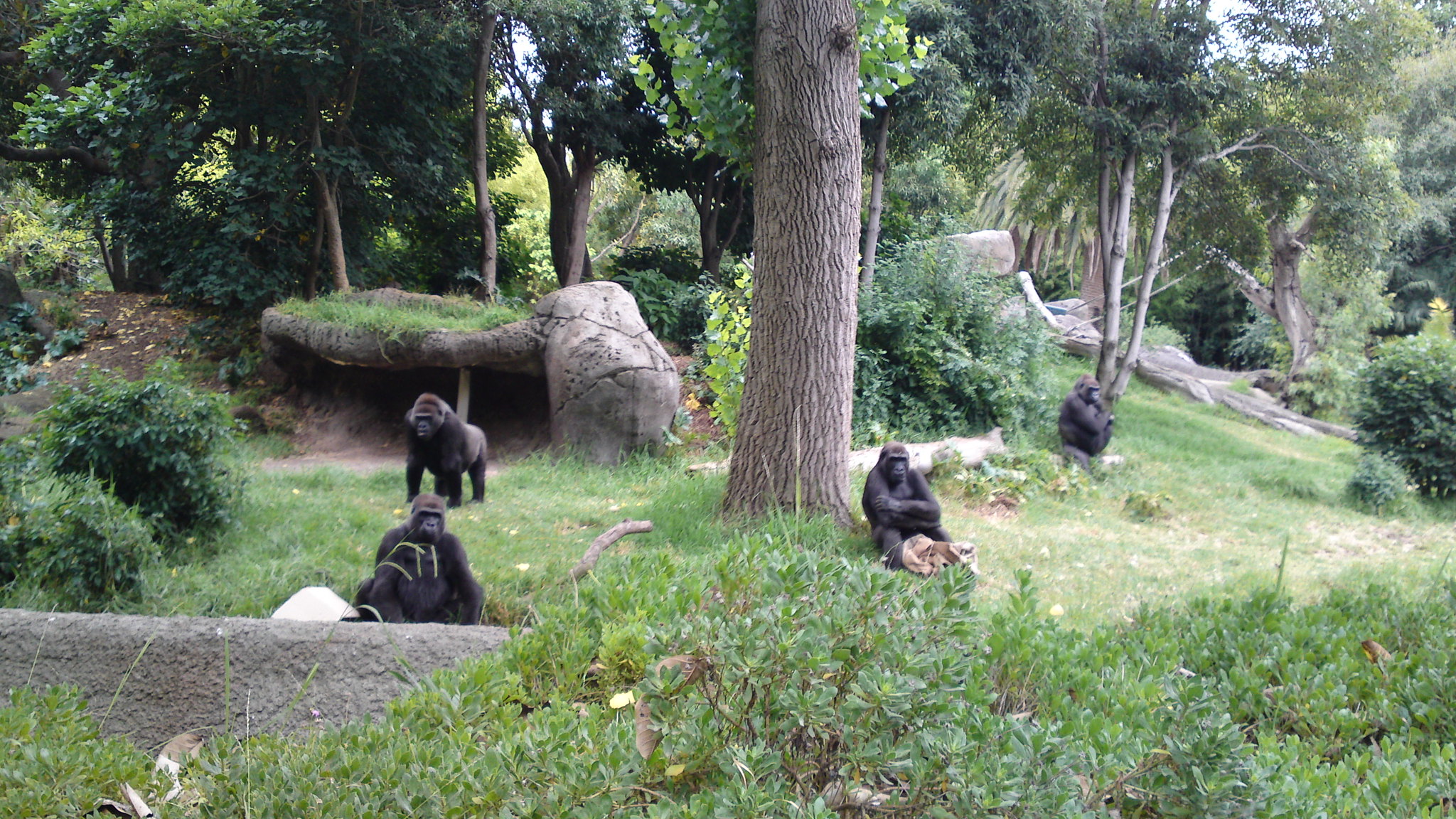In this image, we see a dense, jungle-type setting within a zoo enclosure. The area is filled with a diverse array of very large trees, boasting vibrant green leaves, and various bushes in shades of dark and light green. Prominent gray stones, marked with several cracks, are scattered throughout the terrain. The landscape includes small hills and a little concrete semi-circle wall, adding structure to the scene. Among the foliage and rock formations, there are at least four black gorillas.

In the foreground, one gorilla sits under a tree with its arms crossed, appearing very large and covered in substantial hair. Another gorilla, equally large and imposing, is emerging from behind the concrete wall. Towards the background, a gorilla sits up against a tree, while another, visibly sizable and on all fours, seems poised in a more active stance. Small patches of green grass and little purple flowers add splashes of color to the verdant environment, enhancing the natural beauty of this open, expansive habitat. The overall atmosphere suggests a dynamic yet serene scene, with the gorillas positioned in a way that reflects both their majesty and potentially aggressive demeanor.